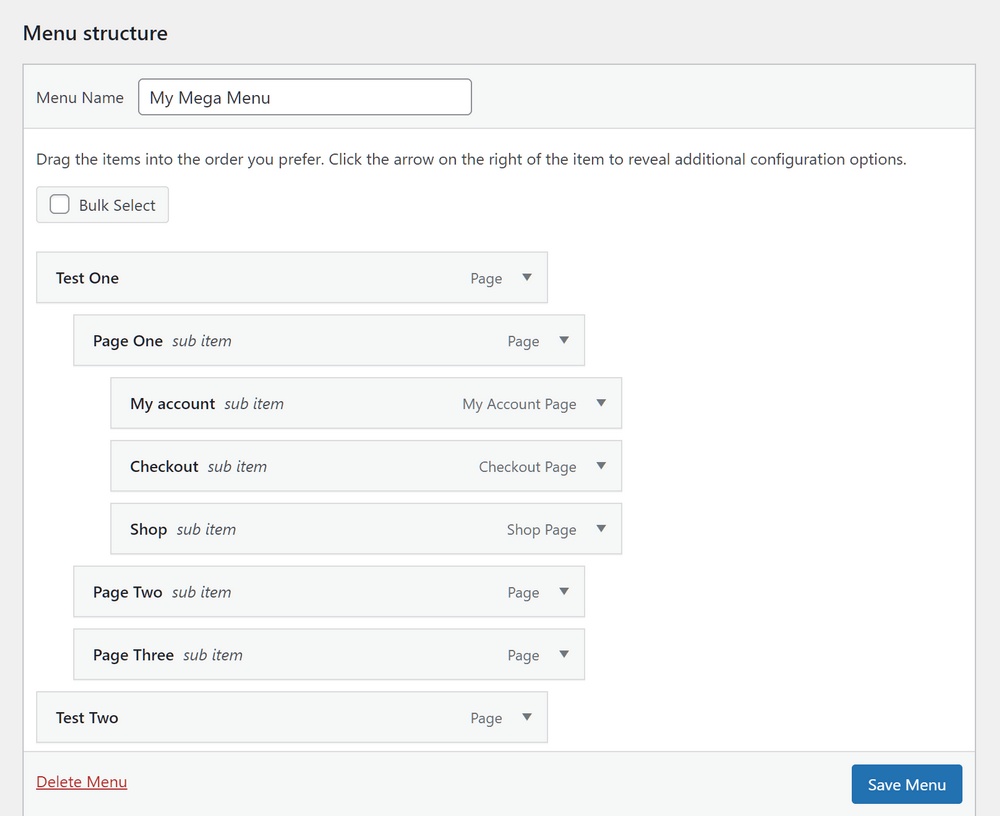The image displays a user interface for configuring a menu structure, set against an off-white (eggshell) background with a white central frame. At the top left, the header "Menu Structure" is presented in black font. Below the header, there is a text box labeled "Menu Name," containing the entry "My Mega Menu." Adjacent to this text box, a search field allows users to input text.

Under the "Menu Name" section, instructive text reads: "Drag the items into the order you prefer. Click the arrow on the right of the item to reveal additional configuration options." Below this instruction, there is a button labeled "Bulk Select" accompanied by a checkbox.

The menu items listed include:
1. Test 1
2. Page 1 (sub-item)
3. My Account (sub-item)
4. Checkout (sub-item)
5. Shop (sub-item)
6. Page 2 (sub-item)
7. Page 3 (sub-item)
8. Test 2

At the very bottom of the interface, there are two options for managing the menu. On the left side, in red font and underlined, the option "Delete Menu" is visible. On the right side, within a blue box, is the "Save Menu" option.